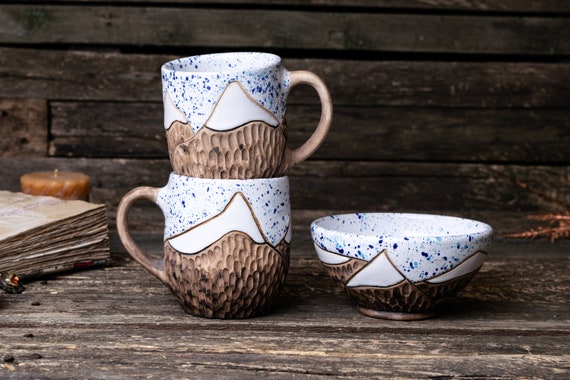The photograph captures a rustic, cozy scene set against what appears to be the interior of an old cabin, characterized by a textured wooden table and possibly a brick background. Central to the image are two ceramic mugs, stacked one atop the other, and a small bowl, neatly arranged and sharing the same intricate, handcrafted design. The ceramics feature a striking pattern: their tops adorned with blue speckles on white, transitioning to a snow-capped white mountain motif over a brown base. The handles of the mugs are a light brown. To the left of these ceramics, there's a small, orange candle beside an older-looking book or a stack of papers, adding a nostalgic touch. On the right, a hint of leaves peeking into the frame enhances the natural, rustic vibe. The wooden table they rest on has seen better days, its worn finish adding character to the setting.